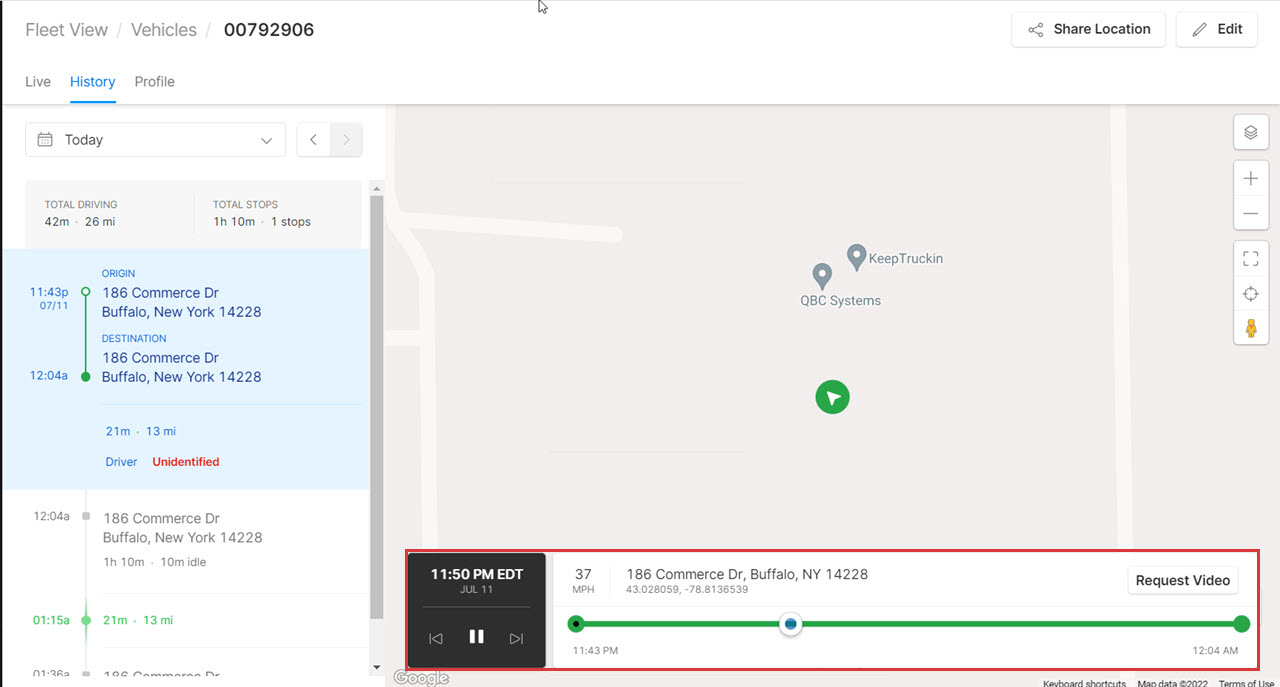This is a detailed screenshot of a vehicle tracking application, presented on a clean, white background. 

At the top left corner, the interface labels are clear: "Fleet View Vehicles" followed by the tracker identification number. Beneath this, the left sidebar features navigation options labeled "Live," "History," and "Profile." Below these options, a drop-down menu marked "Today" allows the user to select specific dates for tracking data.

The detailed information about a specific vehicle is displayed vertically along the left side. This section includes:
- Total driving time: 42 minutes
- Distance covered: 26 miles
- Total stops: 1 stop
- Duration of stop: 1 hour and 10 minutes

Specific timestamps detail the vehicle's journey:
- At 7:43 AM, the vehicle was at a certain address.
- At 12:04 PM, the vehicle was at a different address.

These movements cover 21 minutes and 13 miles, and the driver is noted as "unidentified," marked in red for emphasis.

To the right of this information, a map provides a visual representation of the vehicle's route with pin drops indicating various locations. A round green icon with an angled arrow marks the latest position of the vehicle. At the top right corner of the map, there are controls for zooming in, zooming out, and changing map layers.

At the bottom of the screen, a timeline bar offers playback options with "Rewind," "Pause," and "Fast Forward" buttons, allowing users to review the vehicle's journey. At the right end of this bar, there is an option to request additional video footage from the tracking period.